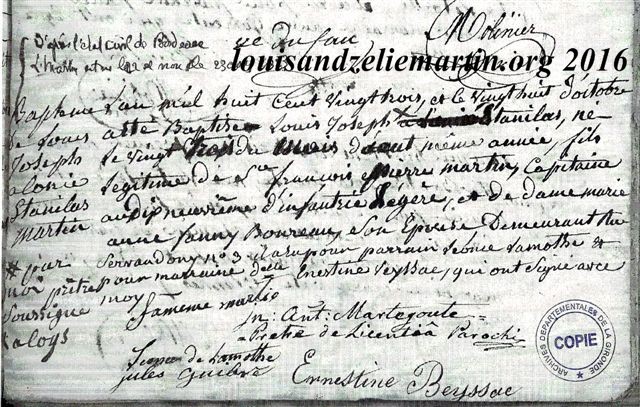This image depicts an aged, historic document written in an old, cursive script, likely with quill pen and ink. The text appears to be in French, as evidenced by the presence of French words and the word "COPIE" (spelled C-O-P-I-E) inside a circular seal in the bottom right corner. The document is signed by several individuals, with the main signature at the bottom belonging to Ernestine Barosi. Other visible names include Jules and different signatures that are hard to decipher. The upper part of the document features printed text stating "Lewis and Zell Martin dot org 2016." The document has a distinctly aged, light gray background with black ink and includes a star at the bottom of the stamp. It appears to be a copy of an important historical text or declaration.